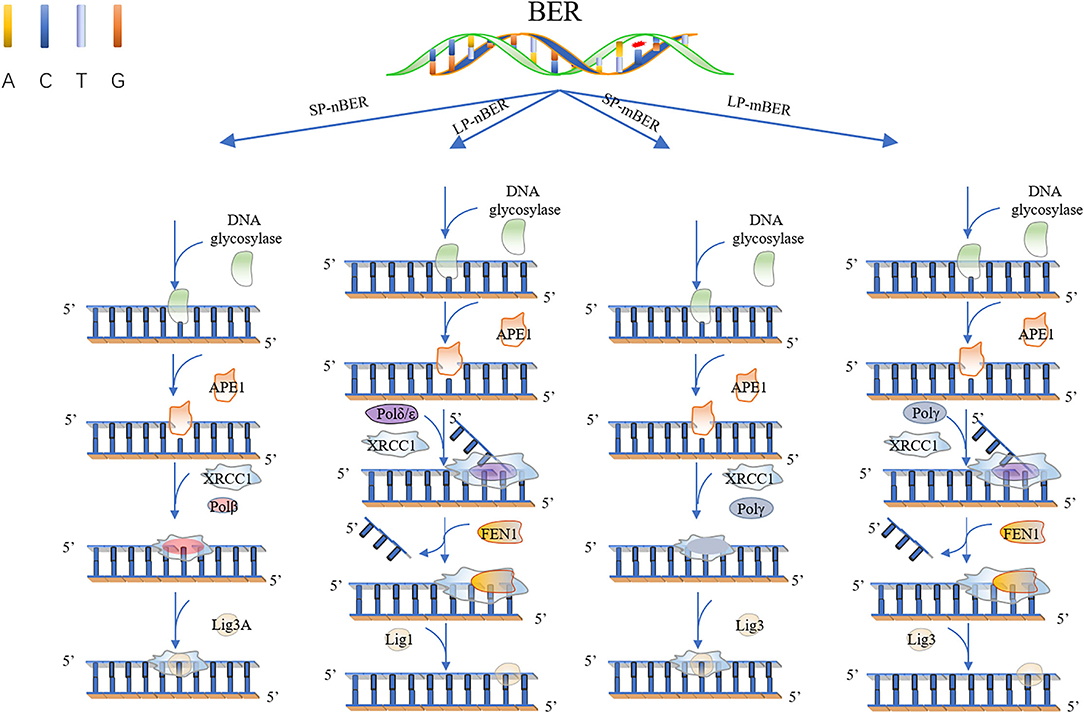This detailed drawing presents a comprehensive illustration of DNA component breakdowns. Rendered in a landscape orientation, the image is centered under the title "BER" (Base Excision Repair). At the top, a twisted DNA strand is displayed, which branches into four distinct groups below.

A clearly marked legend identifies the four DNA bases with corresponding colors: Adenine (A) in yellow, Cytosine (C) in blue, Thymine (T) in gray, and Guanine (G) in red. Each of these bases is strategically represented within the strands.

From left to right, Group 1 and Group 3 contain four DNA strands each, while Group 2 and Group 4 feature five strands apiece. The intricate details of the strands, along with accompanying scientific descriptions, suggest that the drawing is intended for use by scientists or biologists to aid in understanding the nuances of DNA structure and function.